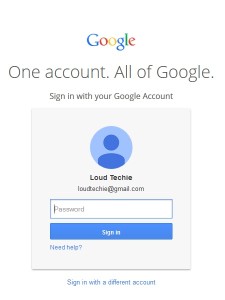The image features a Google sign-in page set against a clean, white background. Positioned prominently near the top center is the iconic Google logo, with each letter rendered in Google's signature colors: blue, red, yellow, blue, green, and red. Below the logo, a prominent slogan in large, light black letters reads, "One account. All of Google." 

Under this slogan, in a smaller gray font, the text instructs, "Sign in with your Google Account." 

A shaded rectangular box contains a round blue icon featuring a generic person symbol, representing the user's avatar. Beside this icon, the username "Loud Techie" is displayed in black, with the associated email address "loudtechie@gmail.com" written directly beneath it in a lighter gray. 

Below the user information, a white banner outlined in blue invites the user to "Enter your password," ensuring the input area is easily identifiable. Further down, a blue button with white lettering says "Sign In." To the left of this button, in smaller blue text, a help link reads "Need help?" with a question mark.

Outside this box, the rest of the page remains predominantly white, with the text "Sign in with a different account" also in blue, positioned towards the bottom of the screen. The overall design is clean and intuitive, with subtle shading to distinguish interactive elements from the background.